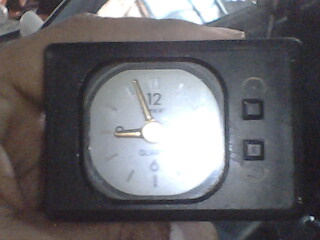In this close-up photo, an old-fashioned, portable alarm clock is held by a person's left hand, with their thumb resting on top and fingers gripping the bottom. The hand, which is white, securely frames the clock, whose outer case is a black rectangle with subtly rounded corners. Inside this outer case lies the actual clock face, also defined as a square with rounded edges. Surrounding the clock face is another black border encasing the mechanism. The clock's face is white, but a bright light casts a glare over nearly half its surface, obstructing some details.

Despite the light, key features remain visible: the numerals 12, 6, and 9 are clearly marked at their respective positions. Though the numeral 3 is obscured, it is likely present, judging by the uniform arrangement. Minimalistic lines indicate the remaining hour positions. Near the top of the clock face, the partially visible letters "Q-U-A" suggest the word "Quartz," and there's an unreadable mark just below the number 12. Adjacent to this white clock face on the black surface are two square buttons, part of the clock's functional design. The background hints at a softly lit room with natural light perhaps streaming through a window, although finer details become indistinct beyond the immediate focus on the clock and the hand holding it.